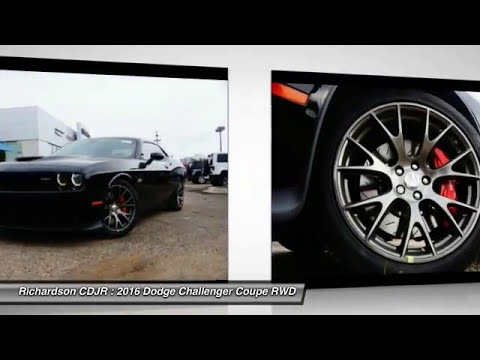The image features two sections displayed on a white wall. On the left, there's a detailed photograph of a black 2016 Dodge Challenger Coupe RWD, parked on paved ground. The car is at a slight angle towards the camera with its wheels turned slightly to the left. Behind the vehicle, there is a black building, other parked cars at an angle, and a bright white sky. The ground in this section appears brown. The right side of the image presents a close-up view of one of the car's tires, highlighting the chrome center with red cables, and part of the vehicle's black body. The entire composition is accompanied by a caption at the bottom which reads, "Richardson CDJR: 2016 Dodge Challenger Coupe RWD."